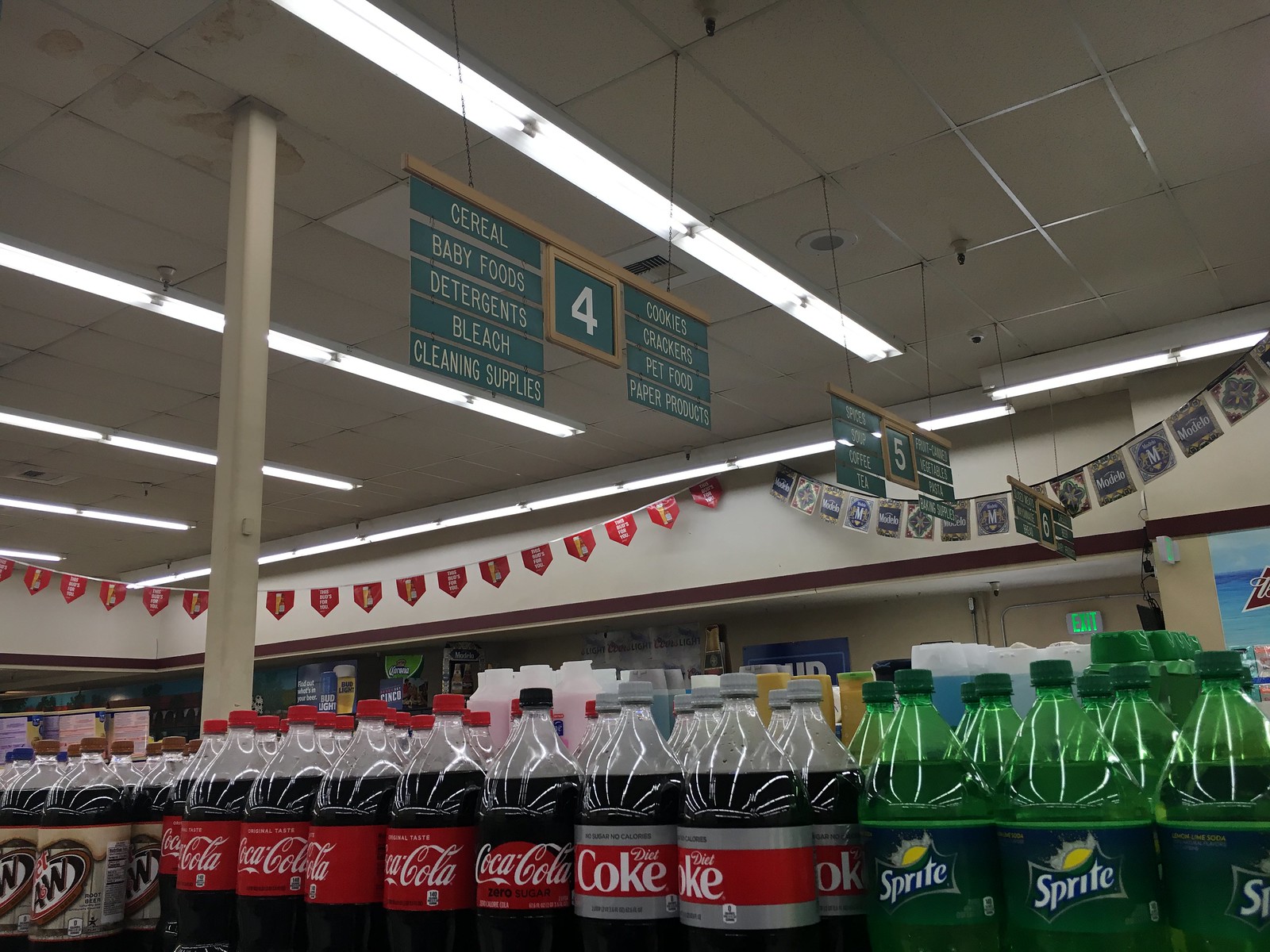This image captures a detailed scene inside a medium-sized supermarket, distinguished by numbered aisles and an organized layout of products. In the foreground, a row of neatly arranged 2-liter soda bottles includes A&W root beer on the left, followed by Coca-Cola, Diet Coke, and green Sprite bottles on the right. Behind the soda bottles, an upright post supports the ceiling on the left-hand side of the image, adjacent to an informational sign indicating aisle 4. This sign, framed in brown with teal blue background and white text, lists categories such as Cereal, Baby Foods, Detergents, Bleach, Cleaning Supplies on the left, and Cookies, Crackers, Pet Food, Paper Products on the right. To the right of this sign, further into the store, is another sign for aisle 5, partially legible with categories like Coffee, Tea, and possibly Vegetables. The background shows a continuation of the store's interior, featuring tiled ceilings with long beams of light, and unclear banners hanging from the upper area, possibly over an open deli or butcher section.